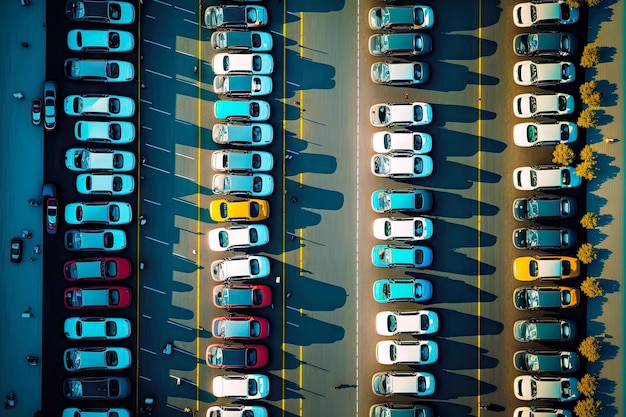This overhead aerial view captures an organized yet dynamic parking lot scene on a sunny day. The parking lot is divided into four distinct rows, each containing various cars parked either forward or backward, aligned in vertical and somewhat scattered arrangements. The cars, which include a mix of small and medium-sized vehicles, come in an array of colors such as white, yellow, red, light blue, and some with two-tone designs like light blue with white roofs. The majority of the cars are electric or of a similar make, creating a visually cohesive display.

In the middle of the parking lot runs an empty road or pathway, serving as the main walking area devoid of moving vehicles. Flanking the parking lot on both the left and right sides are narrow pedestrian walkways. The left walkway is accompanied by smaller vehicles and a few people standing around, while the right walkway features a line of trees with green leaves and some additional pedestrians.

The pavement is marked with yellow and white lines, guiding the parking arrangement. Towards the edges of the parking lot, especially on the right-hand side, there is some noticeable shrubbery casting shadows, contributing to the sunny ambiance of the scene. The overall arrangement and the presence of parked cars imply a well-utilized space, possibly hinting at a busy location frequented by visitors or employees.